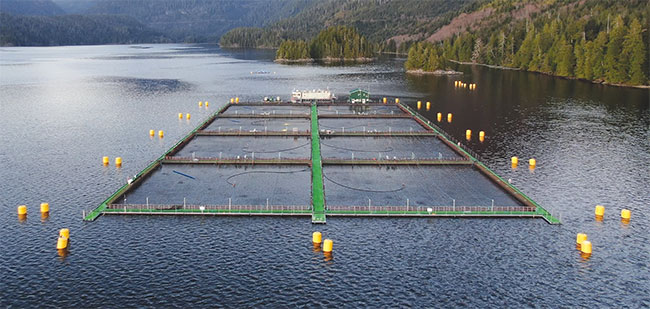This aerial photograph captures a serene lake or river, surrounded by lush green hills and rocky landscapes. The water appears calm and slightly murky, with subtle ripples disturbing its surface. Dotted around the lake are clusters of tall evergreen trees that extend down the slopes and even onto small islands within the water body. Prominently featured in the center of the image is what appears to be a large fish farm or aquatic research facility. This structure consists of a green-painted grid pattern, possibly constructed from metal or wood, floating on the water. It is divided into rows and columns, with walkways outlined in green and some sections covered with nets, indicating active fish farming or some aquaculture activity. The facility is surrounded by numerous yellow buoys, serving both as barriers to keep boats away and markers within the lake. The intricate setup includes lampposts and guardrails for safety and illumination, and two blurred buildings in the background—one green and one white—potentially serve as operational or research stations. This detailed setup indicates a combination of natural beauty and human endeavor towards aquaculture in a mountainous region.